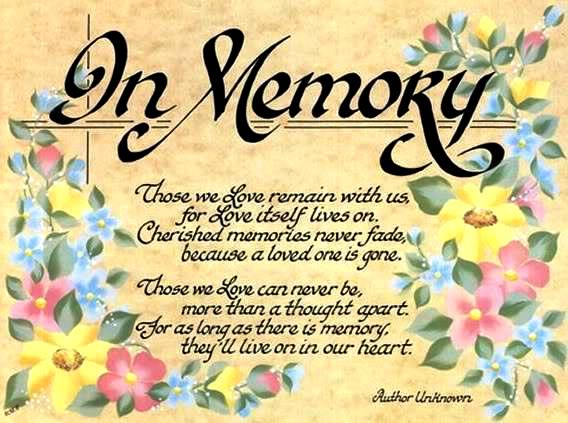The image features a light yellow background adorned with blue, pink, and red flowers along the borders, complemented by green leaves. At the top, in elegant cursive and italicized black letters, it reads "In Memory," with the phrase underlined twice. Below it is a heartfelt poem, also in black italic text, which says:

"Those we love remain with us, for love itself lives on. Cherished memories never fade because the loved one is gone. Those we love can never be more than a thought apart, for as long as there is memory, they'll live on in our heart."

In the bottom right-hand corner, the text "Author Unknown" is noted. A distinctive vertical line intersects the capital 'I' in "In Memory" in the top left-hand section, adding a subtle yet notable detail to this old, memorial-styled card.